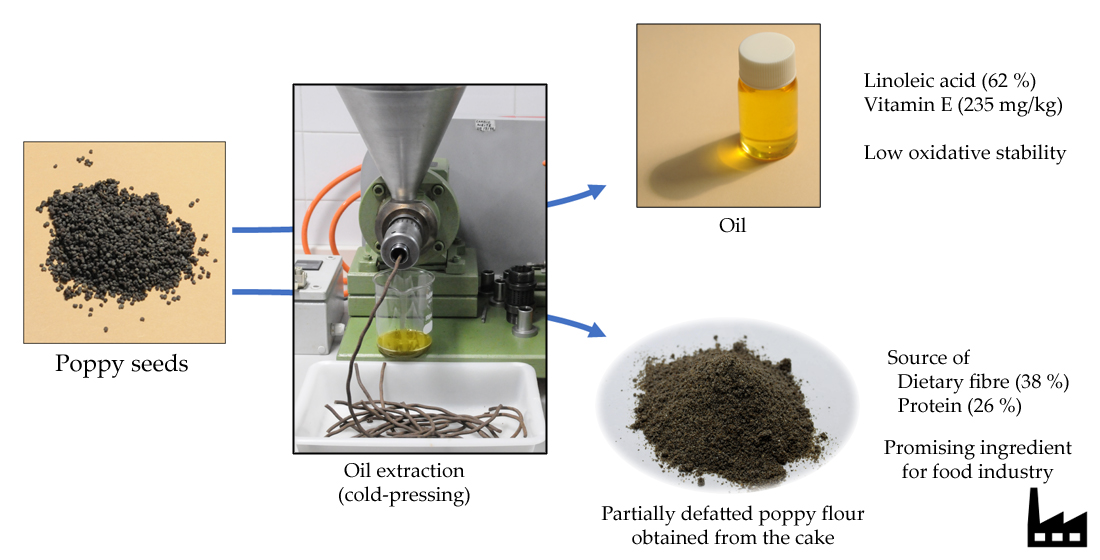The image illustrates a detailed flow diagram of the process for extracting linoleic acid and vitamin E from poppy seeds, using a series of photographs on a white background. Starting from the left, the first photograph features dark brown, almost black poppy seeds labeled "poppy seeds" against a pink background. Blue arrows guide the viewer to the next photograph, which showcases an oil extraction machine conducting cold pressing. This machine extracts oil from the seeds, depicted by a string of liquid flowing into a dish, and simultaneously produces defatted poppy seed pulp into another container.

The arrows then split into two paths. The upper path leads to a small bottle of clear yellow oil with a white cap, displayed on a tan background, labeled with its contents: linoleic acid 62% and vitamin E 235 mg per kilogram. The lower path leads to an image of the partially defatted poppy flour, which is derived from the defatted cake. This flour is highlighted as a promising ingredient for the food industry, rich in dietary fiber (38%) and protein (26%).

Overall, the images and annotations collectively highlight the transformation of poppy seeds into valuable components – oil rich in linoleic acid and vitamin E, and a nutritious defatted flour with significant dietary benefits.